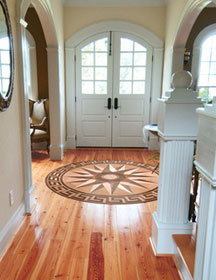This photograph captures the elegant entryway of a luxurious home. The focal point is a set of double French doors painted white, each adorned with black handles. These doors are designed in an arched shape, seamlessly blending into the refined interior. Leading from the front doors, two archways diverge to either side, opening into separate areas of the house. 

The flooring throughout is a shiny, light-colored hardwood, possibly bamboo, with a rich reddish-brown hue. Centered on the floor is a decorative mat that resembles an old nautical compass, featuring shades of brown and orange, perfectly complementing the floor's tones.

To the left, an archway leads into another room, framed by cream-colored walls. A brown mirror with a gold frame hangs on the wall, adding a touch of sophistication. On the right side of the photograph, the initial section of a staircase is visible, characterized by a large pedestal at its base and white stanchions. This captivating entryway sets a grand and inviting tone for the rest of the home.